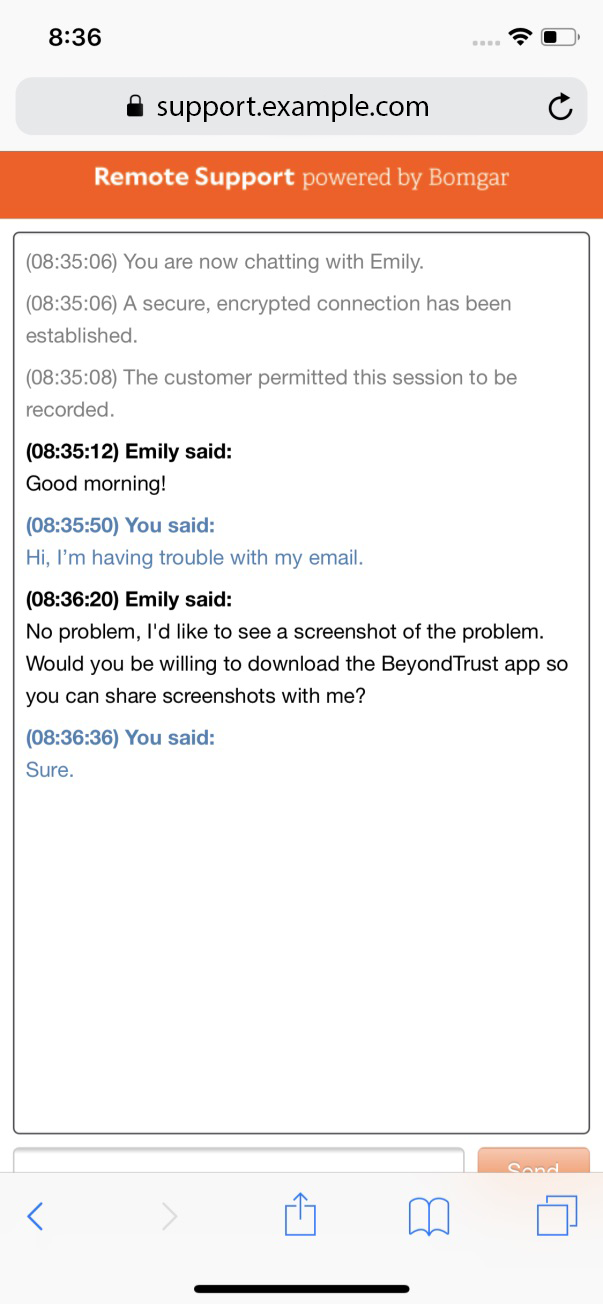In this detailed image caption, we are presented with a screenshot of a technical support chat interface, set against a white background. In the upper left corner, the time is displayed as 8:36. The upper right corner shows four fully lit bars indicating a strong Wi-Fi connection, and the battery icon appears to be half full. Below this, in the address bar, it reads "support.example.com." Directly beneath the address bar is a red strip containing white text that states, "Remote Support Powered by Bomgar."

Below this, the live chat box begins. At 8:35, it notes, "You are now chatting with Emily." Following that, at precisely 8:35 and 6 seconds, a message confirms, "A secure encrypted connection has been established. The customer permitted this session to be recorded." At 8:35 and 12 seconds, Emily greets you with, "Good morning." In response, you state, "Hi. I'm having trouble with my email." Emily replies, "No problem. I'd like to see a screenshot of the problem. Would you be willing to download the BeyondTrust app so you can share screenshots with me?"